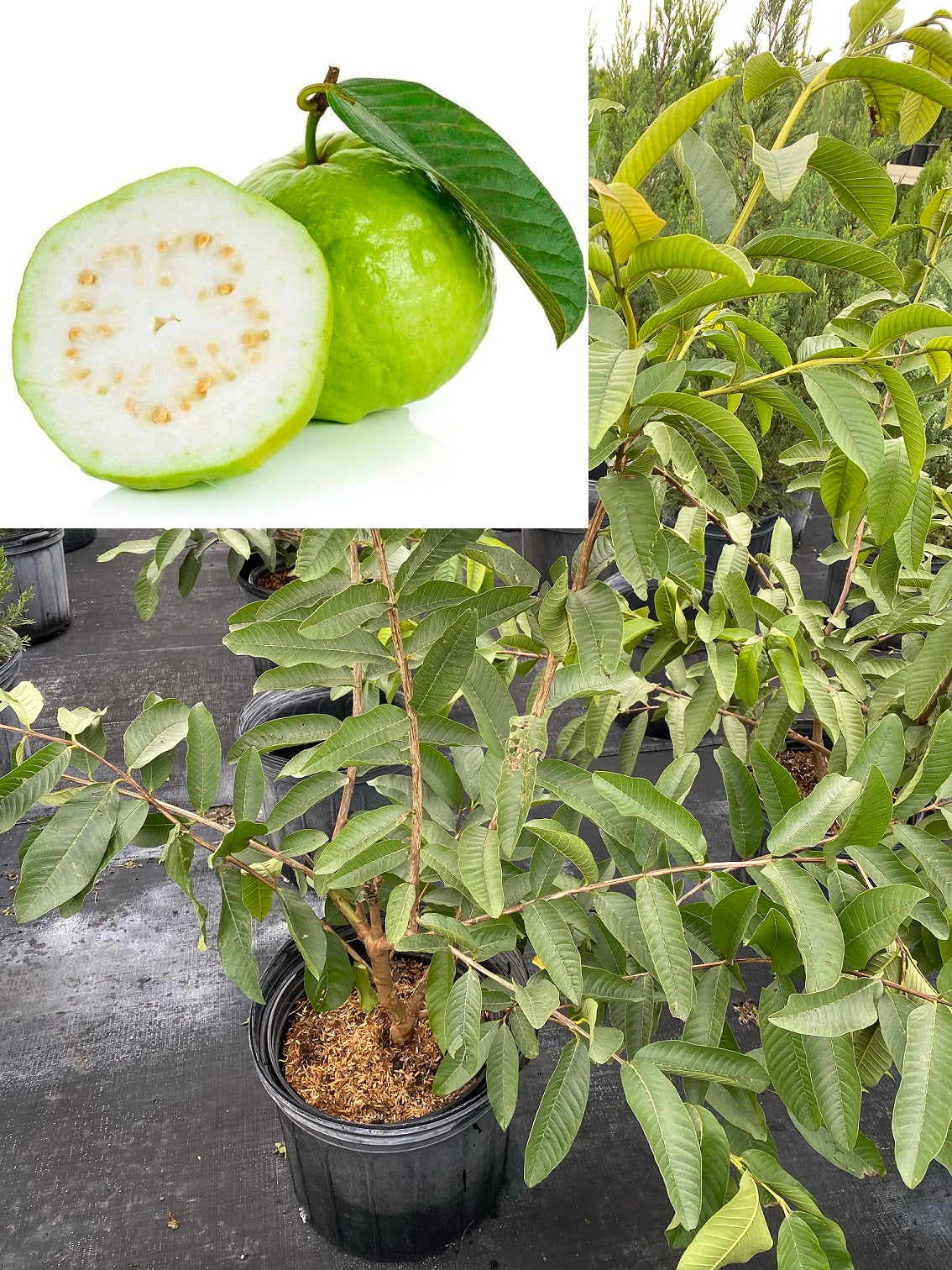The image consists of two photographs, the top left featuring a close-up of a green circular fruit with an attached stem and a large green leaf. One fruit is intact while another is cut in half, displaying its white, pulp-like interior dotted with orange seeds. This half reveals no visible core. The remainder of the image showcases a plant with long, thin leaves akin to those on the fruit, growing in numerous black plastic containers filled with soil. The background suggests a greenhouse setting with other similar potted plants visible, their thin branches and stems intertwining and spreading out in various directions.